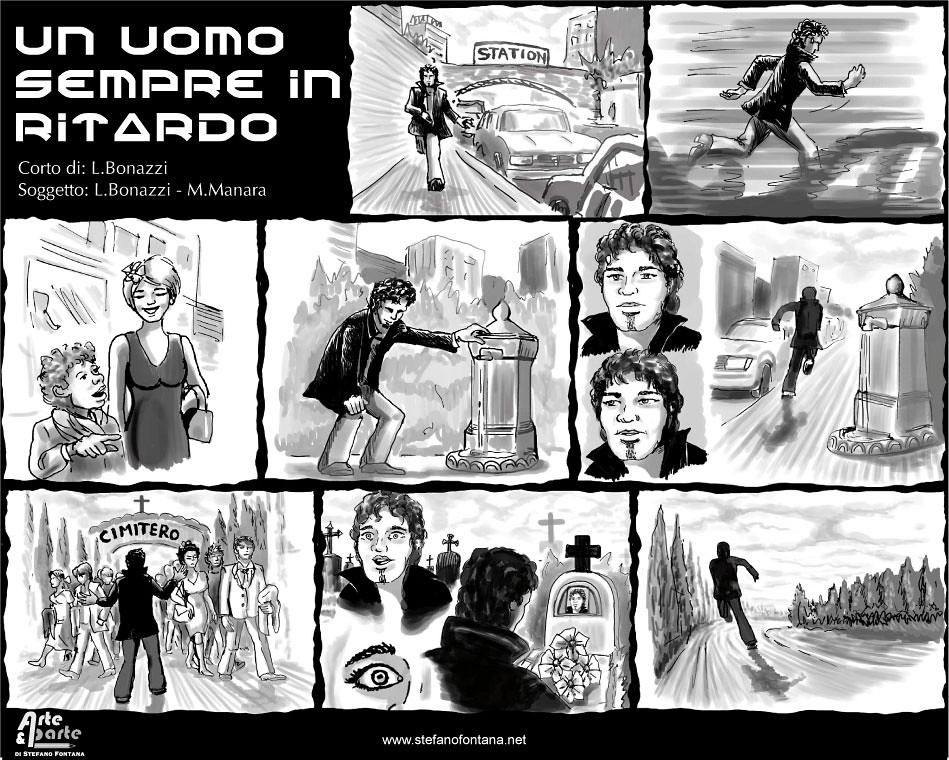This black-and-white, hand-drawn comic-style illustration, titled "Un uomo sempre in ritardo" by L. Bonazzi and M. Manara, is a detailed and narrative-driven artwork. Organized into a 2x3x3 frame layout, the top panels depict a man running alongside a street with the word "Station" prominently displayed, indicating he has missed his intended ride. Moving to the middle frames, we see the character pausing to catch his breath while a woman stands nearby with a child. The subsequent frame continues to show him in motion. Finally, the bottom row dramatically shifts to a cemetery setting labeled "Cemeterio". Here, the man is depicted entering the cemetery as others exit, laying flowers at a gravesite, and then hurriedly leaving. The central figure—a young man with a hip-length black coat, white slacks, and a distinctive goatee—appears both hurried and melancholic, underscoring the story's emotional depth. Further text and credits, including "Corto D. L. Bonazzi" and the website "www.stefanofantana.net", are inscribed throughout the frames, adding context to this poignant and evocative piece.